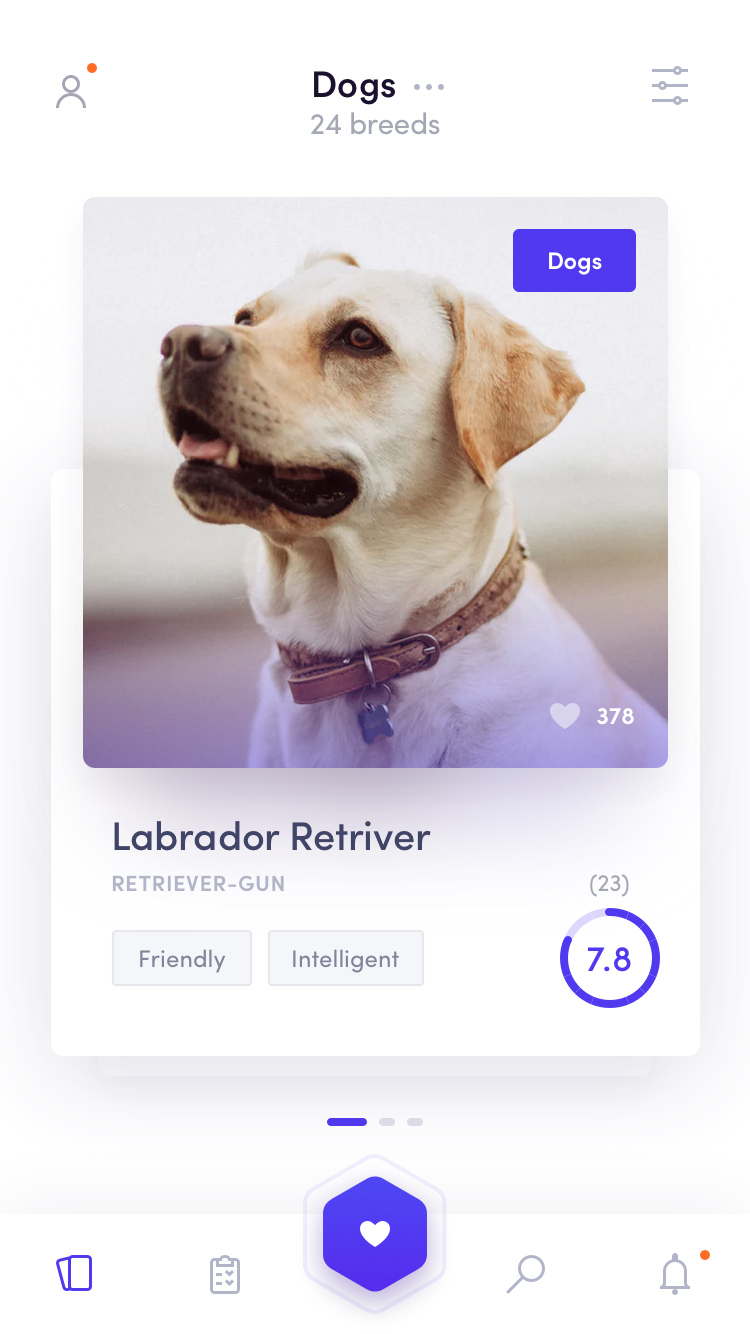**Image Description:**

This is a detailed screenshot from a dog information website. At the top of the page, the heading reads "Dogs," accompanied by a subheading that states "24 Breeds." On the left side of the screen, there's a profile icon. 

The central image features a Labrador Retriever, adorned with a stylish brown leather collar, complete with a silver ring and a name tag shaped like a bone. In the top right-hand corner of this image, a blue button reads "Dogs" in white text. Below it, the text "Labrador Retriever" is highlighted, followed by two descriptors: "Retriever-Gun."

Additionally, there are two grey text boxes underneath the main description, one labeled "Friendly" and the other "Intelligent." A blue circle displaying a rating of "7.8" is also present, alongside a hexagon-shaped icon with a white heart in its center. 

The website appears to be a comprehensive resource for individuals interested in various dog breeds, providing detailed information to help potential pet owners make informed decisions.